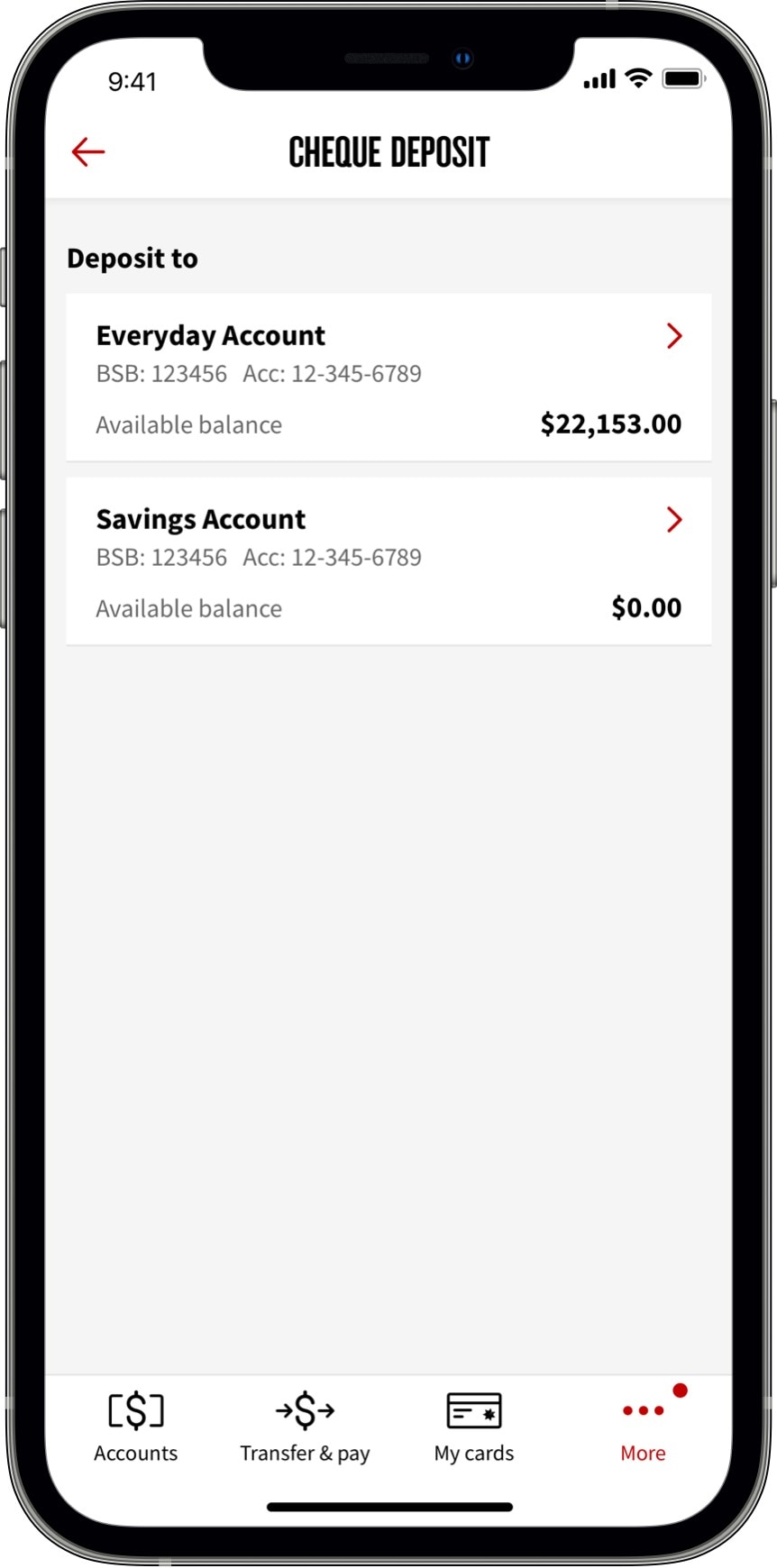The image depicts a smartphone screen with various interface elements and details. The status bar at the top shows the time as 9:41, with full bars of service, Wi-Fi, and battery indicators on the right side.

Below the status bar, the interface presents a "Check deposit" option, labeled as "C-H-E-Q-U-E" in black text, accompanied by a red arrow indicating a back function. Beneath this, the "Deposit to" section is displayed, listing an "Everyday account" in black text with a red arrow on the right.

The account details follow, showing the BSB number, 123456, and the account number, 123456789. The available balance for this account is prominently displayed as $22,153 in black text. An additional "Savings account" option is listed further down, with similar details: BSB 123456 and account number 123456789, but the available balance is shown in gray text as $0.00.

At the bottom of the screen are several options: "Accounts" with a cash symbol inside a box, "Transfer and pay" with a cash symbol and two arrows, "My cards" with an image of a card, all in black text. There are three dots with a smaller dot to the top right, labeled "More" in red text. A black line separates these options from the bottom border of the phone.

The physical appearance of the smartphone includes a black border, a speaker at the top, a front-facing camera lens, and a button on the right-hand side of the phone. On the left side, there are three additional buttons.